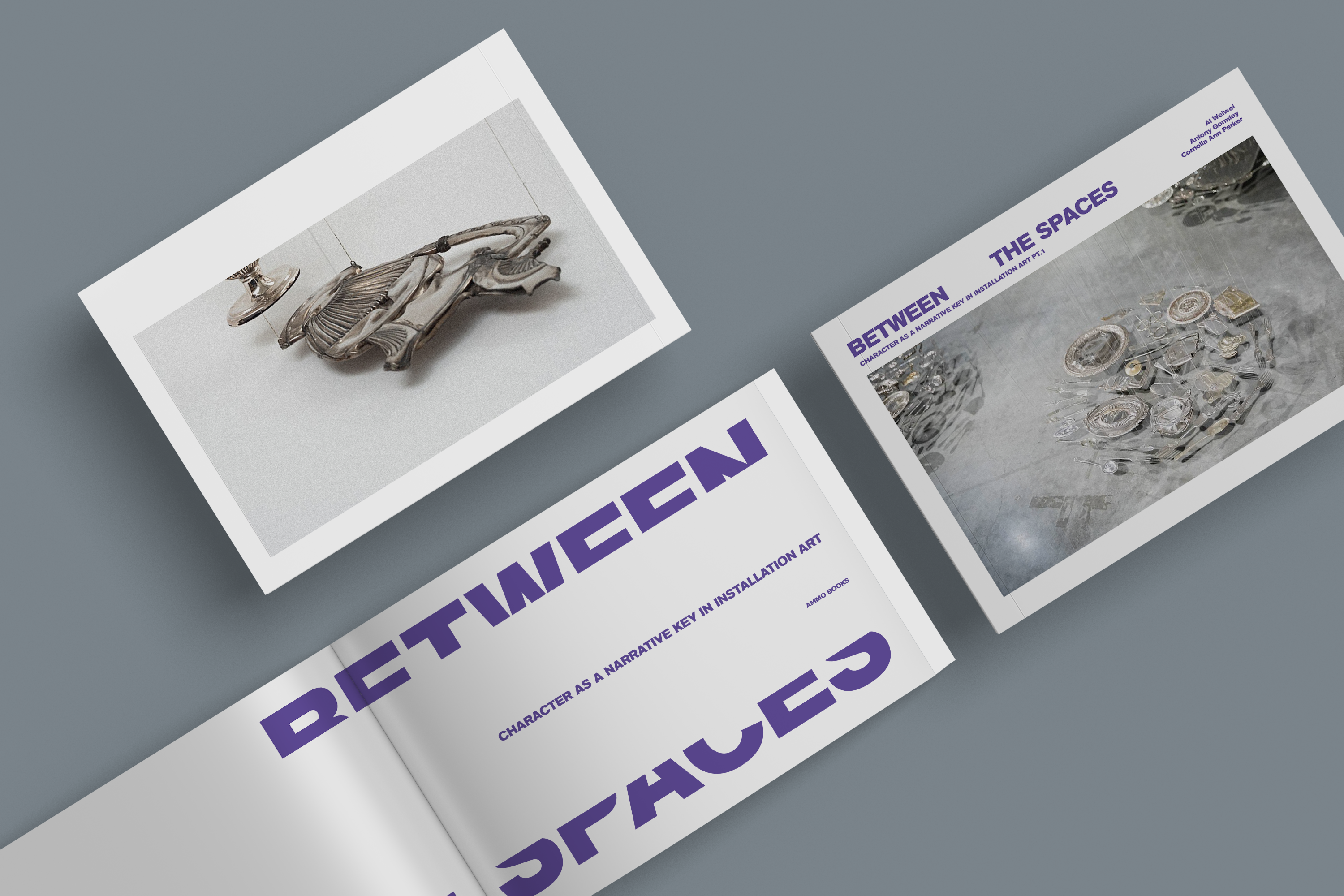The image consists of a digital rendering of a pamphlet and its contents, displayed against a gray background. The pamphlet, printed on white paper stock with prominent purple text, is open to reveal the content. At the top and bottom of the open pamphlet, the words "between" and "spaces" are partially visible, with the text "character as a narrative key in installation art" clearly legible in the center. The pamphlet is from Ammo Books.

Inset within the image are three distinct sections. The upper left section features two metal art pieces. One appears to be the base of a trophy or candle holder, and the other is a long, streaked silver design. Both pieces seem to hang from wires, suggesting they are part of an installation. The upper right section shows multiple plates and silverware arranged in a circular formation, resembling an installation art piece. The lower section showcases the pamphlet's cover, reiterating the text "between the spaces" followed by "character as a narrative key in installation art part one" in purple text.

Overall, the image is a detailed representation of an art installation pamphlet and its featured works, with a focus on silver metallic elements and geometric arrangements.